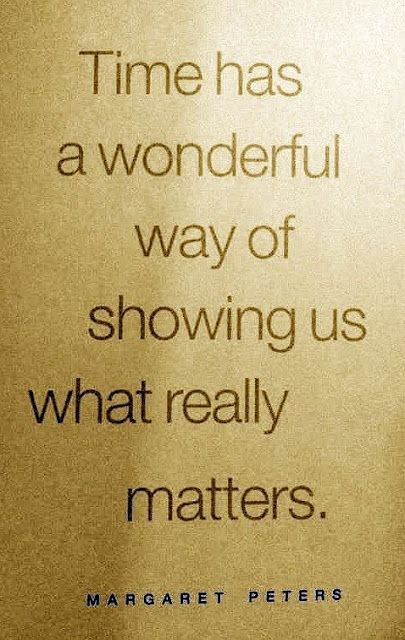The book cover features a tan backdrop resembling the texture of sand, complete with subtle variations in lighting that create a gradient from a brighter top-right corner to a shadowed bottom-left. This elegant cover showcases dark brown text in Times New Roman font, which reads sequentially: "TIME HAS a wonderful way of showing us what really matters." At the very bottom, "Margaret Peters" is prominently displayed in blue, also in Times New Roman. The overall design is straightforward and simple, with the text standing upright and clearly legible against the natural, grainy background.